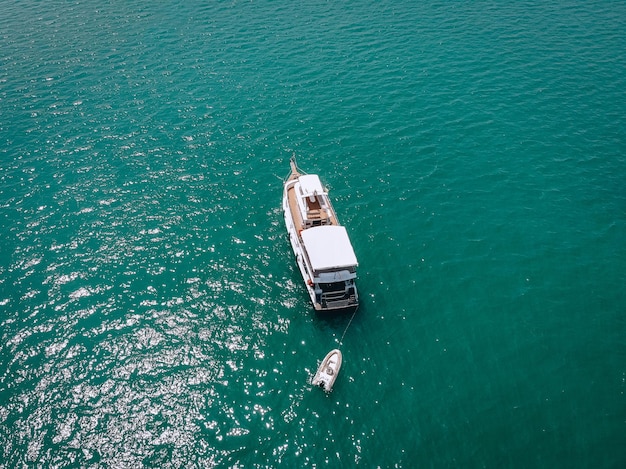This is a detailed aerial, square, full-color photograph taken outdoors during the daytime using natural light, depicting a serene seascape. The background of the image is predominantly water with a greenish aquamarine tint, likely due to algae. The water is calm and reflective, with sunlight shimmering particularly in the lower right-hand corner and along the left side.

At the center of the photograph are two boats. The larger vessel is a white double-decker or triple-decker yacht with a brown deck, appearing to head out to sea. This boat generates a visual sense of movement, heading towards an open exploration. Attached to the back of this yacht via a line is a smaller, white rubber dinghy, suitable for one or two people, commonly referred to as a life raft. 

Together, the boats are portrayed elegantly against the tranquil, sunlit water, creating a scenic and inviting depiction of a leisurely or potentially fishing expedition on a beautiful, sunny day.